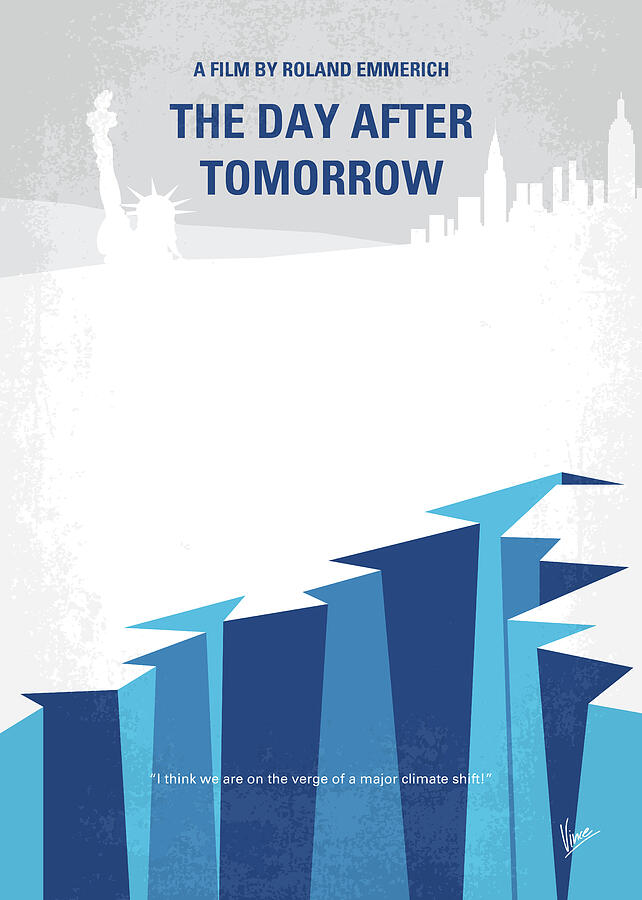The movie poster for "The Day After Tomorrow," directed by Roland Emmerich, features a stark and minimalistic color palette of white, gray, and various shades of blue. The top portion of the poster has a mottled gray background with the title "The Day After Tomorrow," and the text "A Film by Roland Emmerich" written in blue lettering. A white expanse dominates the center of the poster, overlaid faintly with the silhouettes of the New York City skyline on the right and the iconic Statue of Liberty's head and arm on the left. This white area transitions into a menacing, jagged blue cliff or crevasse towards the bottom, symbolizing an icy landscape fraught with peril. Below this icy chasm, near the bottom right-hand corner, there is a quoted text in white letters that reads, "I think we are on the verge of a major climate shift," possibly signed by someone whose name starts with the letter "V." The overall design creates a sense of imminent threat and environmental upheaval, mirroring the film's theme of a catastrophic climate event.